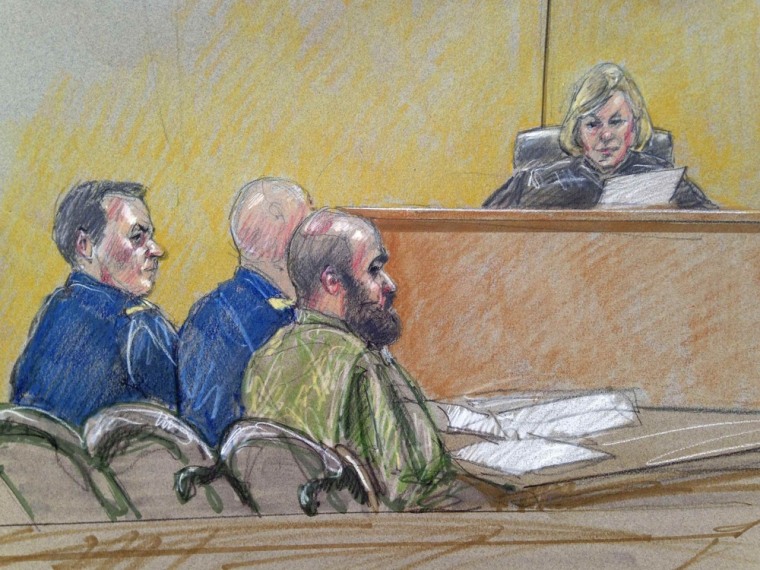The image depicts a colored courtroom sketch, illustrating a tense scene during a court trial. The sketch, executed in a loose style using colored pencil or pastel, captures the essential elements of the courtroom scenario. At the center, a female judge, with short blonde hair styled in a bob, is seated at her bench, wearing traditional black judge's robes. She appears distressed as she reads a piece of paper, her gaze directed downwards at the individuals before her.

In front of the judge, three men are seated at a table cluttered with various pieces of paperwork. The man in the middle, presumably the defendant, wears an olive drab green outfit and has a bald head with a very full black beard. His expression is one of deep concern as he looks off into the distance. Flanking him on either side are two uniformed officers. The officer to his left wears a matching blue outfit with what resembles a badge on his shoulder, and he has a crew cut with brown hair. The officer to the right is bald, also in a similar blue uniform, possibly signifying a military or police rank. His facial expression is stern, glaring intently at the defendant, while the other officer's face is partially obscured but appears to be looking forward towards the judge. 

Overall, the sketch vividly conveys the tension and formality of the courtroom scene, focusing on the expressions and posture of the key figures involved.